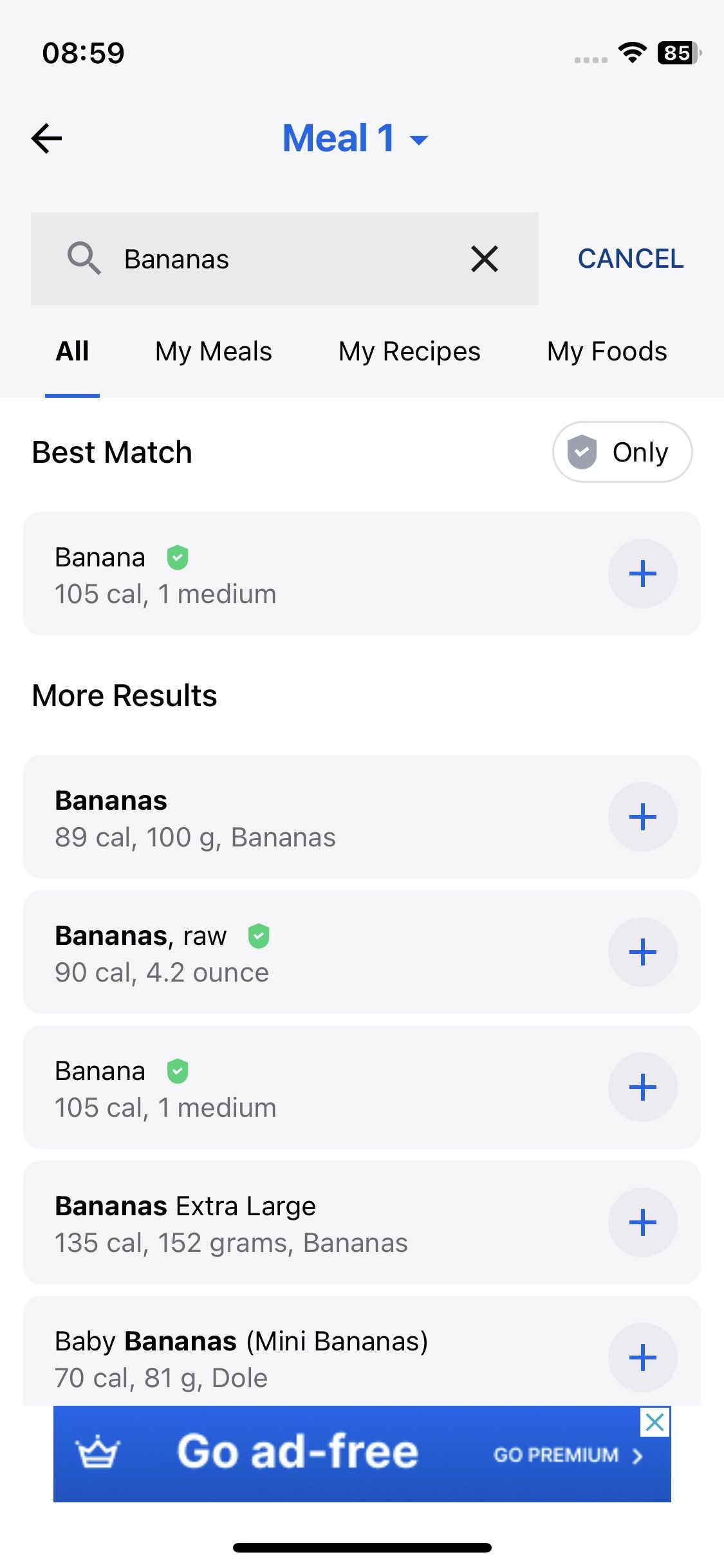The image appears to be a detailed screenshot from a food tracking application. At the top, the status bar displays the Wi-Fi symbol, a battery icon indicating 85%, and the time as 8:59. The main screen has a predominantly white background with black text, and at the top, a blue text label reads "Meal 1" with a dropdown arrow beside it.

Beneath the header is a search box containing a magnifying glass icon. The text "bananas" has been typed into the search field, accompanied by a black "X" to clear the entry and a blue "Cancel" button. Below the search box is a bar listing options: "All", "My Meals", "My Recipes", and "My Foods", with "All" highlighted by a blue underline.

The first search result is titled "Best Match" for "banana", marked with a green icon. It lists nutritional information as "104 cal, one medium", and includes a blue circular plus sign for adding the item. Subsequent results include "Bananas" (89 cal, 100g), "Bananas raw" (90 cal, 4.2 oz), "Banana" (105 cal, one medium), "Bananas extra-large" (135 cal, 152g), and "Baby bananas (mini bananas)" (70 cal, 81g), among others. Each item also features a green icon and can be added via a blue plus sign.

At the bottom of the screen, a blue box with a crown icon and white text offers a premium, ad-free version of the app. The box contains a "Go Ad-Free, Go Premium" message, along with a blue "X" to close the offer. A thin black line runs below this promotional box.